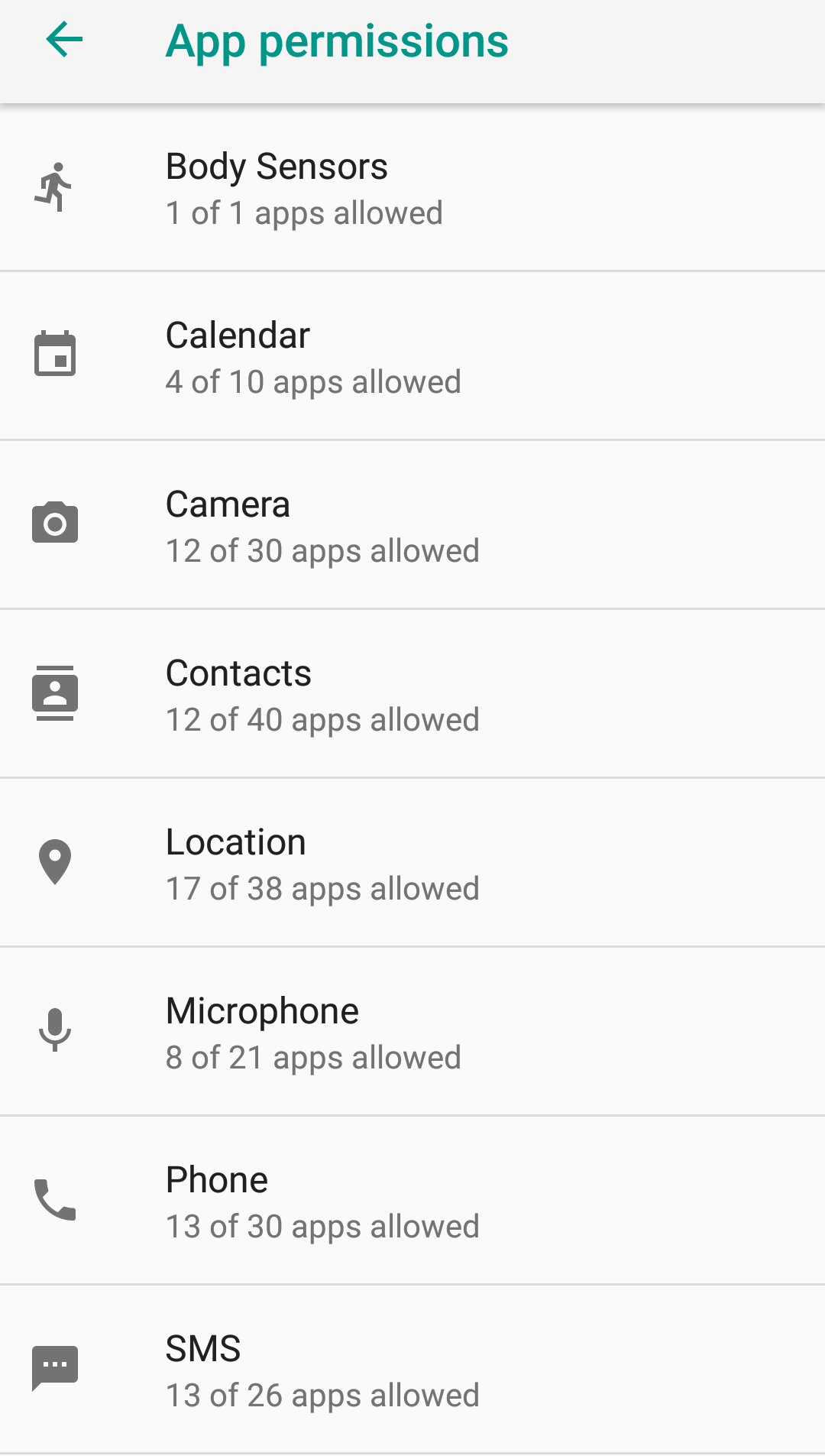This digital image displays a detailed overview of app permissions on a device, organized with icons, text, and specific data points. At the top left corner, there is a back navigation arrow. The page begins with the category "Body Sensors," highlighted by a gray stick figure running icon, with information indicating that 1 out of 1 apps are allowed. Following this, the "Calendar" section is introduced, featuring a gray and white calendar icon, and notes that 4 out of 10 apps have permission to access this feature.

Continuing down the list, the "Camera" section appears next, marked by a gray and white camera icon, and shows that 12 out of 30 apps have camera access. After that, the "Contacts" section is mentioned, indicating that 12 out of 40 apps are permitted, although no additional icon or image is detailed here. Similarly, the "Location" section is described next, with a digital pin icon accompanying it, showing that 17 out of 38 apps are allowed access.

Further down, the "Microphone" section specifies that 8 out of 21 apps are allowed, without an accompanying icon. The "Phone" section reports that 13 out of 30 apps have permission, and the "SMS" section concludes the list, indicating that 13 out of 26 apps are allowed, though no icons are described for these last two sections. The entire image emphasizes the structured organization of app permissions on the device, visually represented through icons and numerical data.